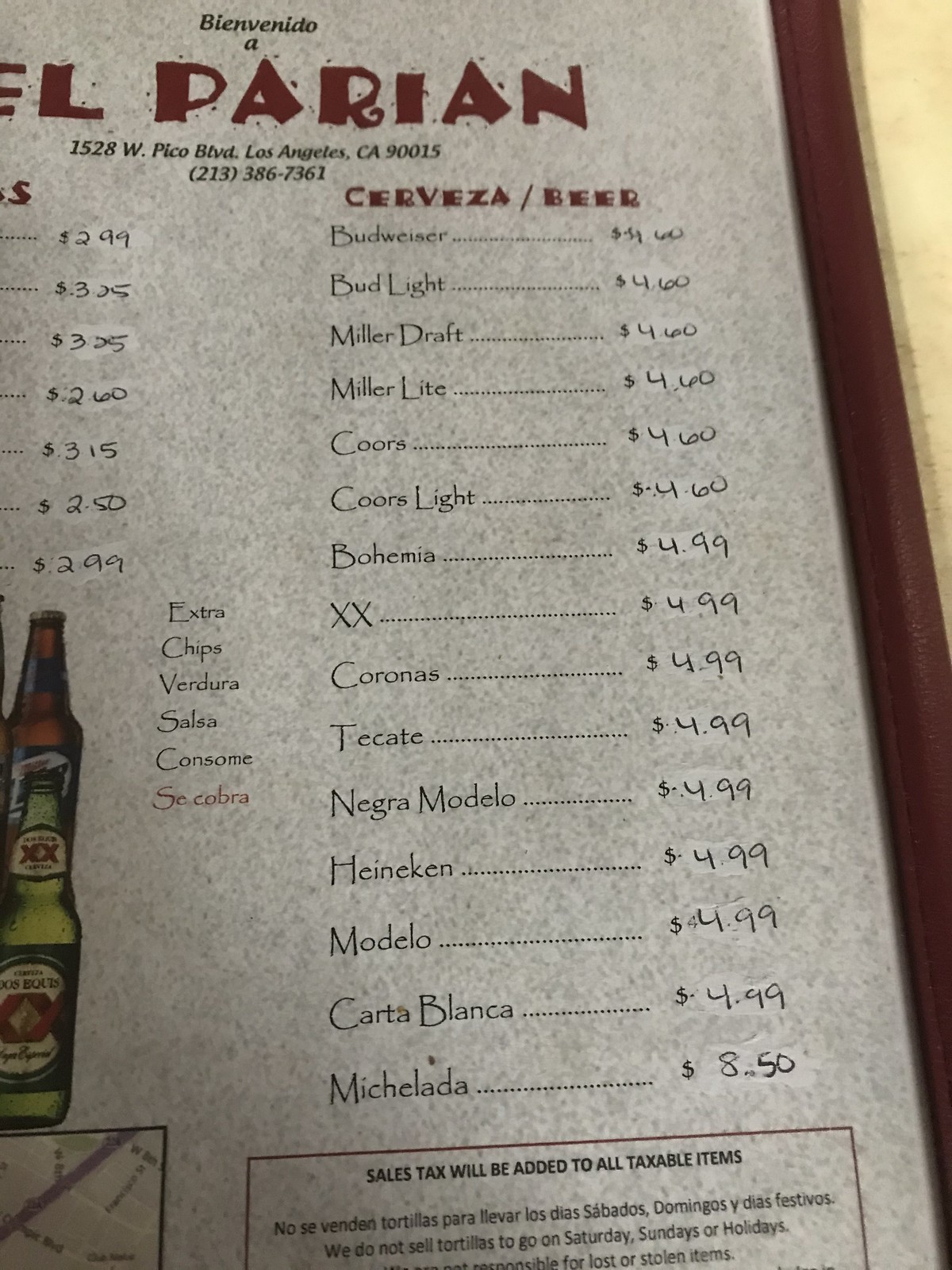This photograph captures a close-up of the drink section of a menu, specifically focusing on the alcoholic beer options. The menu appears to be either hung on a wall or part of a handheld menu from a restaurant. Dominating the top of the image, in bold maroon block letters, is the name "El Patián." Beneath it, in smaller black print, the address "1528 West Pico Boulevard, Los Angeles, California, 90015" is listed, followed by the phone number "(213) 386-7361" in black text.

The menu page, set against a gray background designed to mimic a stony texture, features the title "Cerveza/Beer" in red print. Below this title, a list of beers is presented in a black papyrus typeface. Each beer name is followed by hand-written prices inscribed in black pen. The beers listed from top to bottom are: Budweiser, Bud Light, Miller Draft, Miller Light, Coors, Coors Light, Bohemia, XX, Coronas, Tecate, Negra Modelo, Heineken, Modelo, Carta Blanca, and Michelada.

At the very bottom of the page, partially cut off, there is a message in black text stating, "Sales tax will be added to all taxable items." Below this, a note in Spanish reads: "No se venden tortillas para llevar los días sábados, domingos, y días festivos," which translates to "We do not sell tortillas to-go on Saturdays, Sundays, or holidays."